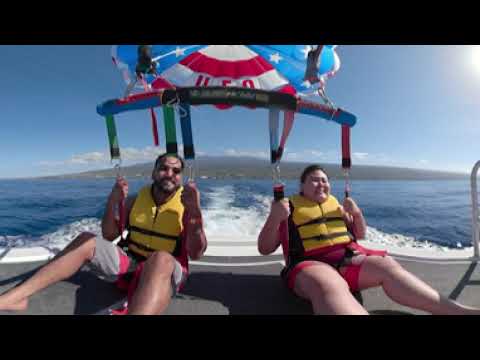In an outdoor setting with a vast body of water, possibly a lake or the ocean, a man and a woman are seated on the edge of a gray boat, ready for parasailing. Both are wearing yellow life jackets. The man, with dark hair, a goatee, and dressed in gray shorts, is positioned on the left. The woman, also with dark hair and wearing red shorts, is on the right. Each holds onto harnesses connected to a large parachute above, designed to resemble the American flag with blue, red, and white stripes, white stars, and the word "UFO" emblazoned on it. The boat leaves a wake in the water, suggesting movement, and the sky above is blue with a few clouds. In the distance, there are scenic mountains, an island with some houses, and an expanse of water all around. Both individuals are smiling in anticipation as they prepare to be lifted into the air.